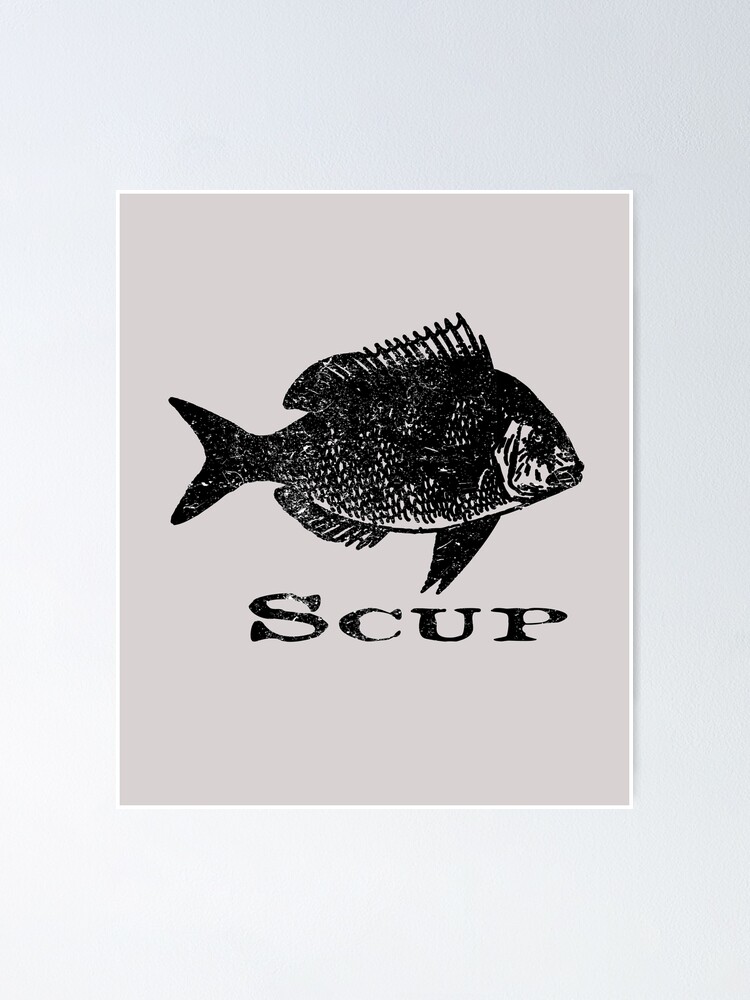The image features a black-and-white fish with a somewhat bored facial expression, positioned on a vertically aligned, cream-colored rectangle set against a white border. The fish's body transitions from a predominantly black color to a lighter gray on the underside, with notably sharp and spiky fins. Below the fish, the single word "scup" is written in capital letters, "S-C-U-P," in a black, screen-printed style font. The overall aesthetic of the image has a hand-drawn, screen printing texture, contributing to its detailed and textured appearance.